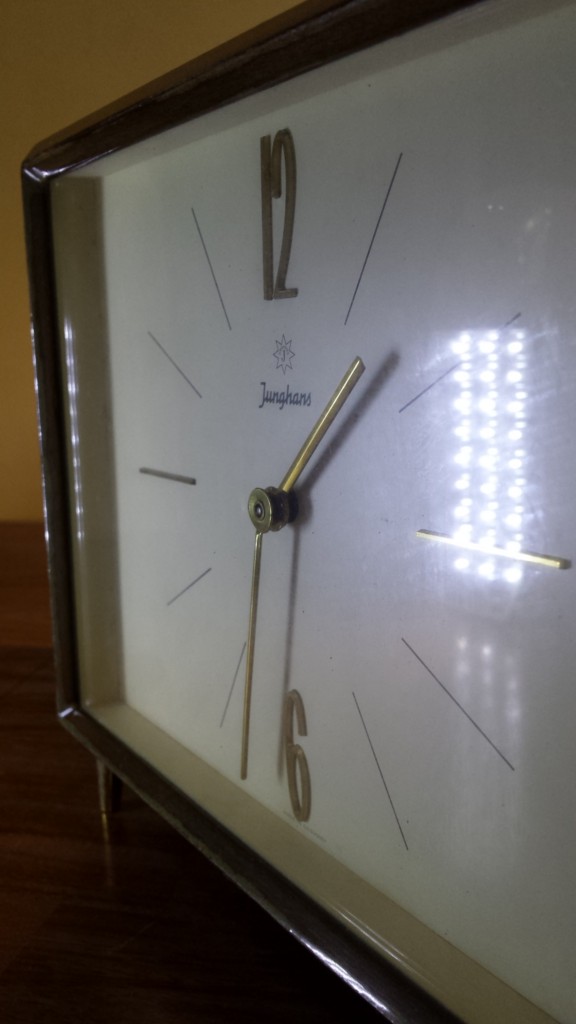This is a detailed close-up photograph of a vintage or antique clock, likely positioned on a dark wooden desk or table. The clock, square in shape, features a white face framed by a cream-colored border set within a black enamel or ceramic case. Prominently displayed on the clock face are the gold numbers "12" and "6," positioned at the top and bottom center, respectively. The remaining hours are indicated by thinner gold lines. The clock hands, which are simple linear gold sticks without arrows, point to approximately 1:30. Above the clock hands, and beneath the "12," the logo "J-U-N-G-H-A-N-S" is elegantly inscribed in a cursive font. Additionally, there are reflections visible on the clock face, including the shadows of the clock hands and what appears to be the bright light filtering through a glass block door or window across the room. The clock stands on short, stubby legs, adding to its classic and refined aesthetic.